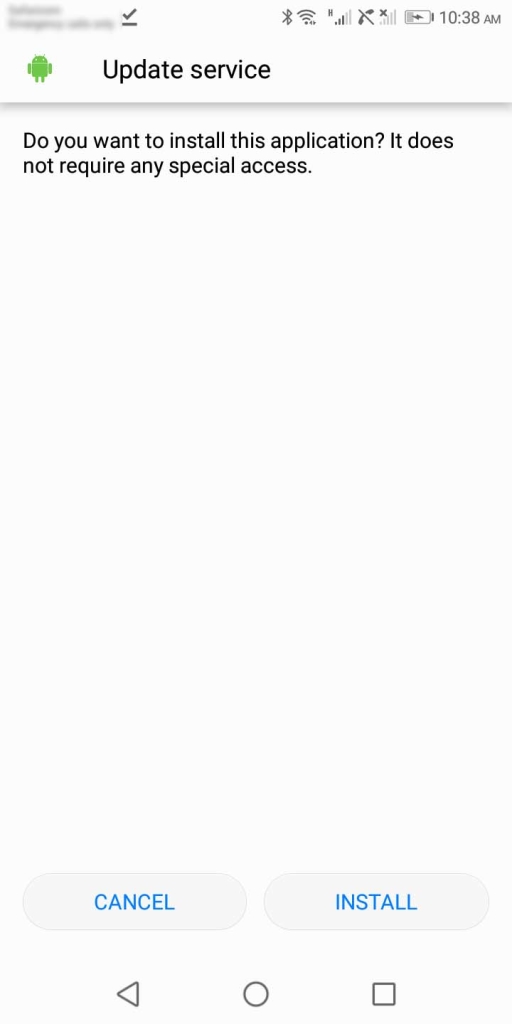A screenshot of a mobile device window displays a prompt for an application update. At the top, the title "Update Service" is accompanied by a green robot icon on the left. Below the title, the text "Do you want to install this application? It does not require any special access." is clearly visible. The main body of the message is blank, showing a plain white screen. At the bottom, there are two buttons: "Cancel" on the left and "Install" on the right.